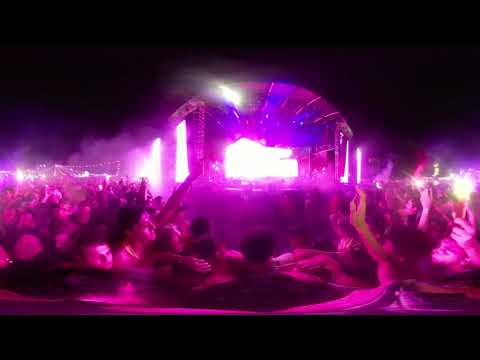The photograph is a very blurry image of what seems to be a concert or performance setting, bathed in rich hues of purple, pink, and blue. The top part of the image is completely black, creating a stark contrast against the vibrant, neon lights below. Dominating the middle section of the image is a tall, arched stage structure, illuminated with bright white lights at its center, which cast a smoky haze of pink into the air. 

Two columns are distinguishable, with beams of light shining through, adding to the ethereal atmosphere. The lighting extends to both sides of the stage, blending the neon pink and purple hues with the surrounding area. The scene below is jam-packed with a crowd, making the ground appear densely populated with heads, hands, and raised arms, all reflecting the purple and pink glow. People's faces are indistinct due to the blurriness, but most of them are seen from the back, focused intently on the stage. In the lower left foreground, one individual stands out, facing right in profile with shoulder-length dark hair, possibly of Caucasian descent, seated and adding to the atmosphere of anticipation and energy.